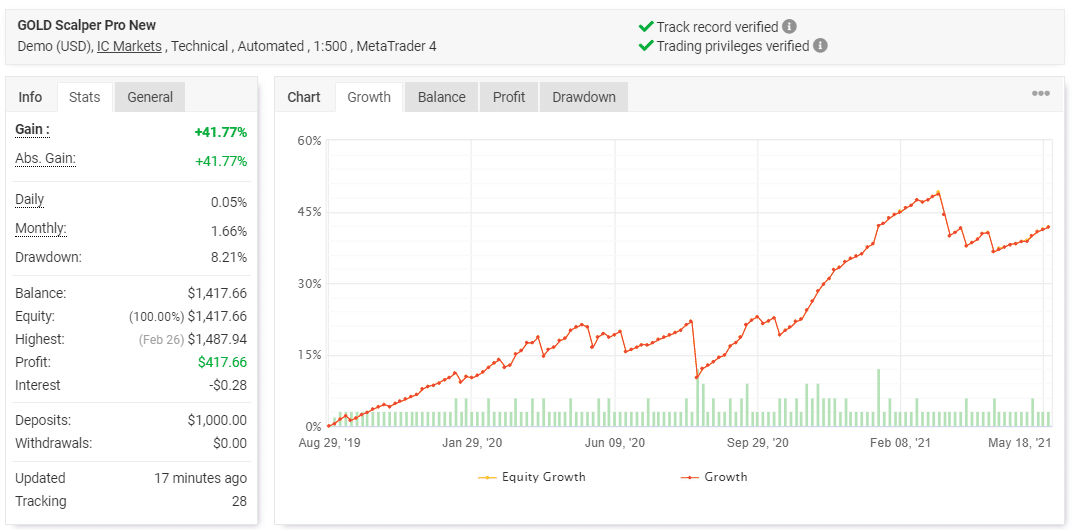The image displays a detailed chart tracking the growth of a financial asset, likely a stock. At the top of the chart, the title reads "Gold Scalper Pro New," followed by "Demo (USD), IC Markets, Technical, Automated, 1:500, MetaTrader 4" in smaller text. Verified check marks indicate both "Track Record Verified" and "Trading Privileges Verified."

On the left-hand sidebar, there are several tabs labeled "Info," "Stats," and "General," with the "Stats" tab currently selected. This tab displays various metrics including the percentage of gains over different time periods, as well as the balances, equities, profits, deposits, and withdrawals in dollar amounts. It also shows the frequency of updates and tracking duration.

In the main section of the image, an X-Y axis chart is prominently featured. The Y-axis, labeled in percentages, ranges from 0% at the bottom to 60% at the top, indicating growth. The X-axis displays dates from August 2019 to May 2021. A red dotted line traces the performance of the asset, showing fluctuations but indicating an overall upward growth trend over the specified time period.